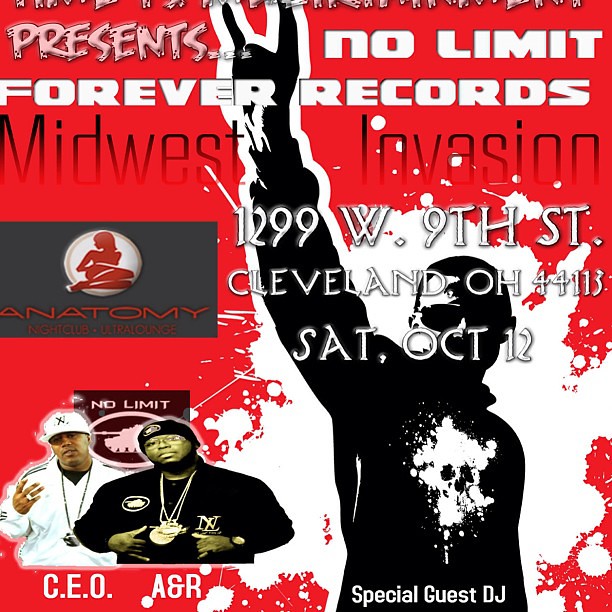This is a professionally designed advertisement for a musical event titled "No Limit Forever Records Midwest Invasion" set to take place at 1299 West 9th Street, Cleveland, Ohio, 44113 on Saturday, October 12th. The sign predominantly features a black and white silhouette of a person, presumably a special guest DJ, making the "rock on" hand gesture and wearing sunglasses. The background includes a mix of black, white, red, and brown colors with white paint splatter effects. At the lower-left corner, there are images of two African American men wearing chains and hats: one labeled as "CEO" and dressed in white, and the other labeled as "A&R" and dressed in black. This visually striking, yet minimalist, poster serves to promote the upcoming musical event.